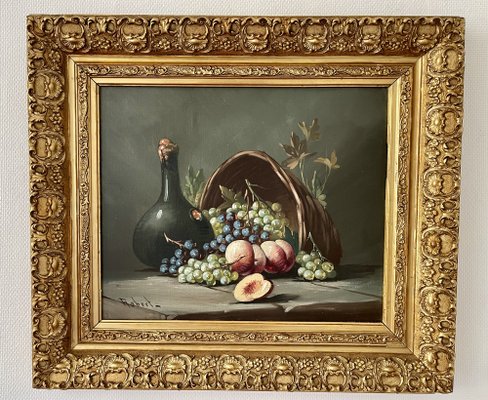This photograph showcases an exquisitely detailed oil painting set indoors, mounted on a white wall. The focal point of the painting is a cornucopia-like basket, tipped on its side to reveal an abundance of green and black grapes spilling out. Situated in front of the basket are several brownish fruits, one notably cut open to expose its gouged-out pit, likely suggesting they are stone fruits. To the left of the basket sits a wide, green wine bottle with a wax-sealed top. The basket and bottle rest on a stone ledge, with flowers subtly peeking out from behind. The painting is encased in an ornate, gold frame rich with curly cues and intricate designs, further surrounded by an even thicker, highly decorative outer frame, weaving a repetitive carved pattern. The scene is set against a gray wall, devoid of any text, allowing the artwork's vibrant palette—comprising various shades of green, purple, brown, black, gray, and the golden hue of the frame—to stand out splendidly.